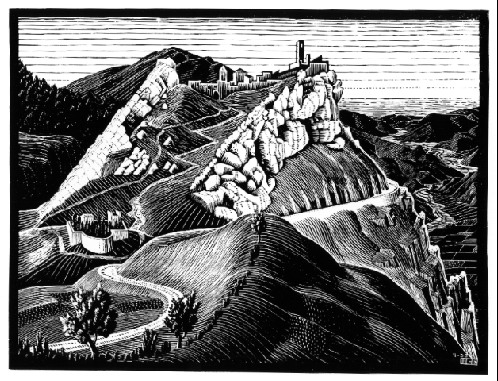This is a small horizontal rectangular black and white painting, depicting an intricate and surreal landscape. In the foreground, a craggy and majestic mountain features a winding road that starts from the bottom left and curves to the right, disappearing into the distance. The mountain's texture is rendered in a charcoal-black color, giving it a dramatic and imposing presence. To the right of this road, an odd outcropping resembling stone appears, adding to the surreal quality of the scene.

Behind this primary mountain, a secondary form emerges, intriguingly shaped like the head and neck of a horse. Adjacent to it, another similar shape, though less realistic, gives the illusion of a second horse. Further back, another large dark mountain looms, its sides adorned with peculiar white, squishy shapes that resemble fungus.

In the left part of the image, towering structures suggestive of a high-altitude city or castle rise, featuring tall, squared-topped buildings and various other structures. To the left of these buildings, a zigzagging road or conduit cuts through the landscape.

In the distant background, a river or creek meanders to the right, past additional mountain ranges that extend towards the horizon. The sky above these mountains is depicted with expansive horizontal and dotted lines, creating an impression of an open, cloud-covered expanse. The combination of finely lined detailing and surreal elements crafts an enigmatic and captivating visual narrative.